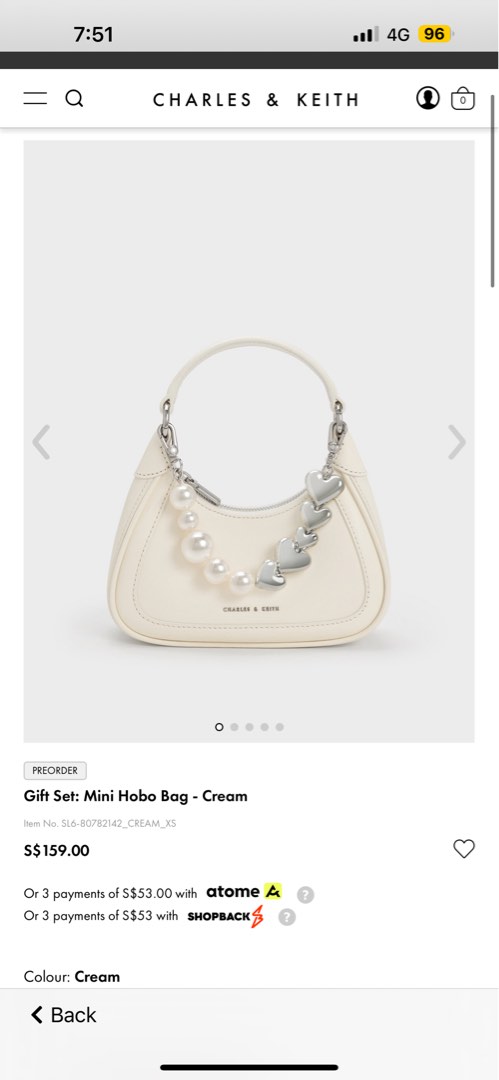Screenshot of a Charles and Keith Online Store Product Page

This image captures a screenshot from the Charles and Keith online store. Displayed prominently at the top center is the product name "Gift Set: Mini Hobo Bag in Cream." The bag, depicted in the image, is white with a distinctive chain strap. The left side of the chain features elegantly designed pearls, while the right side consists of charming silver hearts.

The price of the bag is listed as $159, denoted by an 'S' symbol followed by a dollar sign: S $159. Below the price, there are payment options mentioned for pre-order: "Three payments of $53 with Atome" or "Three payments of $53 with Shopback." The text also reaffirms the bag's color as cream.

Additional interface elements in the screenshot include a back button located at the bottom left corner. At the very top of the screenshot, the status bar reveals the time as 7:51 AM on the left. On the right side, the phone's signal strength shows three out of four bars, it is connected to a 4G network, and the battery is at 96% with the Low Power Mode icon displayed.

Overall, the detailed presentation aims to provide a comprehensive view of the product and relevant purchase options for potential customers.